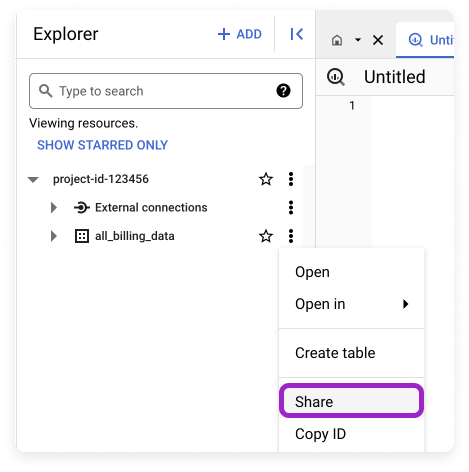The image depicts a web page layout with a clean, organized interface. Centered on an all-white background, the layout begins at the top with the text "Explorer" in dark black font. Beneath this header is a plus symbol followed by the word "ADD" in capital letters. Adjacent to this is a left-facing arrow icon.

Further down, there is a search box marked by a magnifying glass icon and the prompt "type to search." To the right of this search box is a question mark enclosed in a black circle.

Below this search area, more white space follows, displaying the text "Viewing resources, show star only," highlighted in blue. There's a drop-down menu labeled "project-ID-123456" accompanied by a star icon and a vertical ellipsis (three vertical dots).

Next, there is a right-facing arrow icon beside the label "External connections," which also features a vertical ellipsis. 

Further down, more options are listed with the text "all," which is underlined, followed by "billing," and "data," each also underlined. This section concludes with another vertical ellipsis.

In the subsequent column, an entry marked "Untitled" is followed by the number 1. Superimposed on this section is a rectangle featuring options such as "open," "open in," "create table," and "share," the latter of which is outlined in purple. Lastly, the option "copy ID" completes the layout.